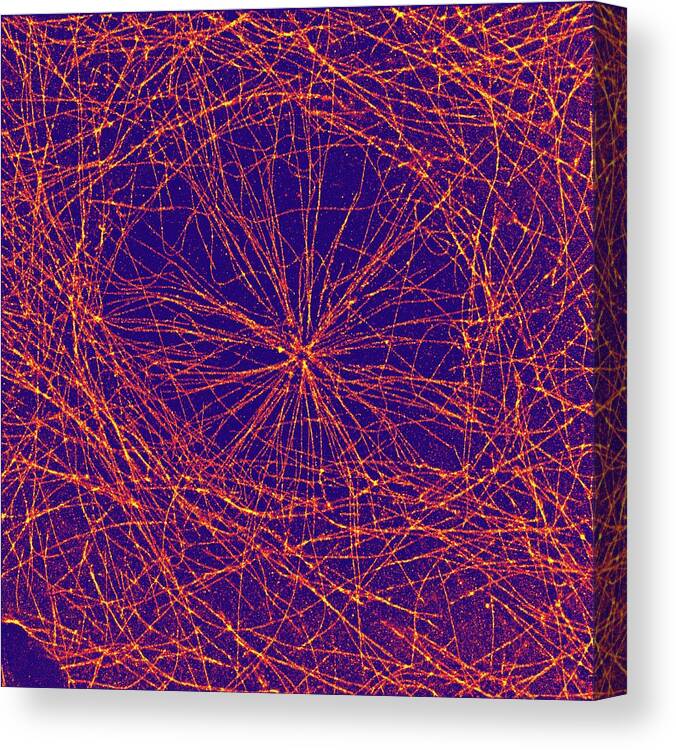This abstract work of art features a striking royal blue, almost purple, matte canvas as its background. The canvas exhibits a dynamic, interlacing spiderweb-like pattern comprised of thin, spiraling lines that range in color from reddish-orange to pink, with occasional neon yellow highlights. The intricate design starts from the center of the canvas and radiates outward in a star shape, revolving around itself to form a nest-like structure. The right edge of the canvas, visible from the angle of the photograph, adds a 3D quality to the piece, with the colorful lines appearing to drip off the side. Shadows and variations in the richness of color on different parts of the canvas further enhance its textured, multi-dimensional appearance. The entirety of the vibrant blue background is covered with the haphazardly crisscrossing lines, resulting in a visually captivating and richly detailed abstract piece.